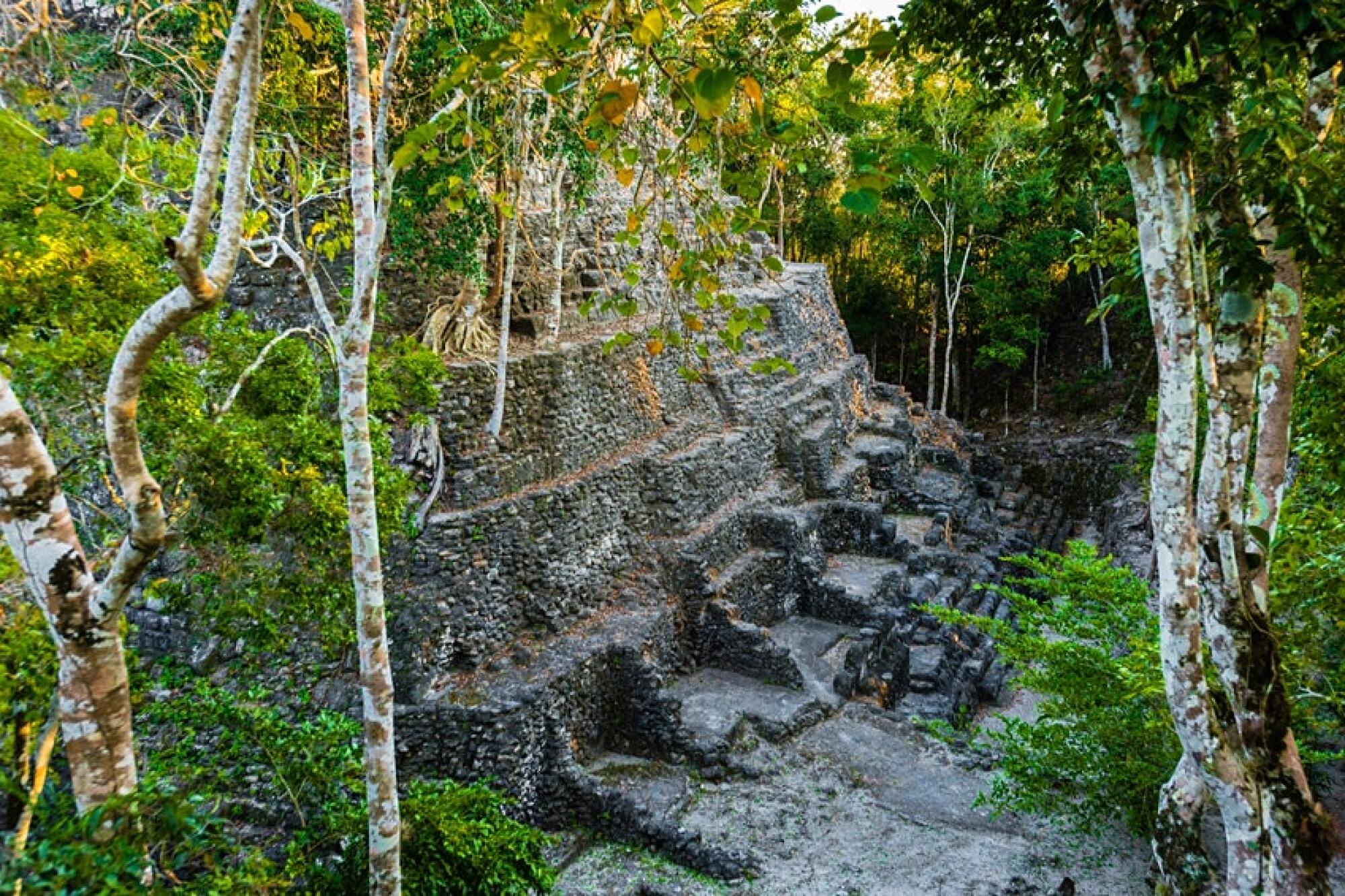This color photograph, taken from a high vantage point, features an ancient Mayan pyramid-like temple set amidst a lush jungle. The structure, which appears to be centuries old, is constructed entirely from hand-stacked stone bricks, giving it a terraced appearance with at least four visible levels. Stone staircases are prominent at the base and in the middle of the structure, with the surrounding higher ground suggesting it may be partly dug into the earth. The temple has a crumbling, aged appearance, surrounded by towering green trees with white and brown trunks on both sides and more vegetation in the background. Sunlight filters through the tree tops, illuminating the scene with a natural glow. The image is devoid of any people, animals, or motorized vehicles, leaving the ancient, serene setting undisturbed.